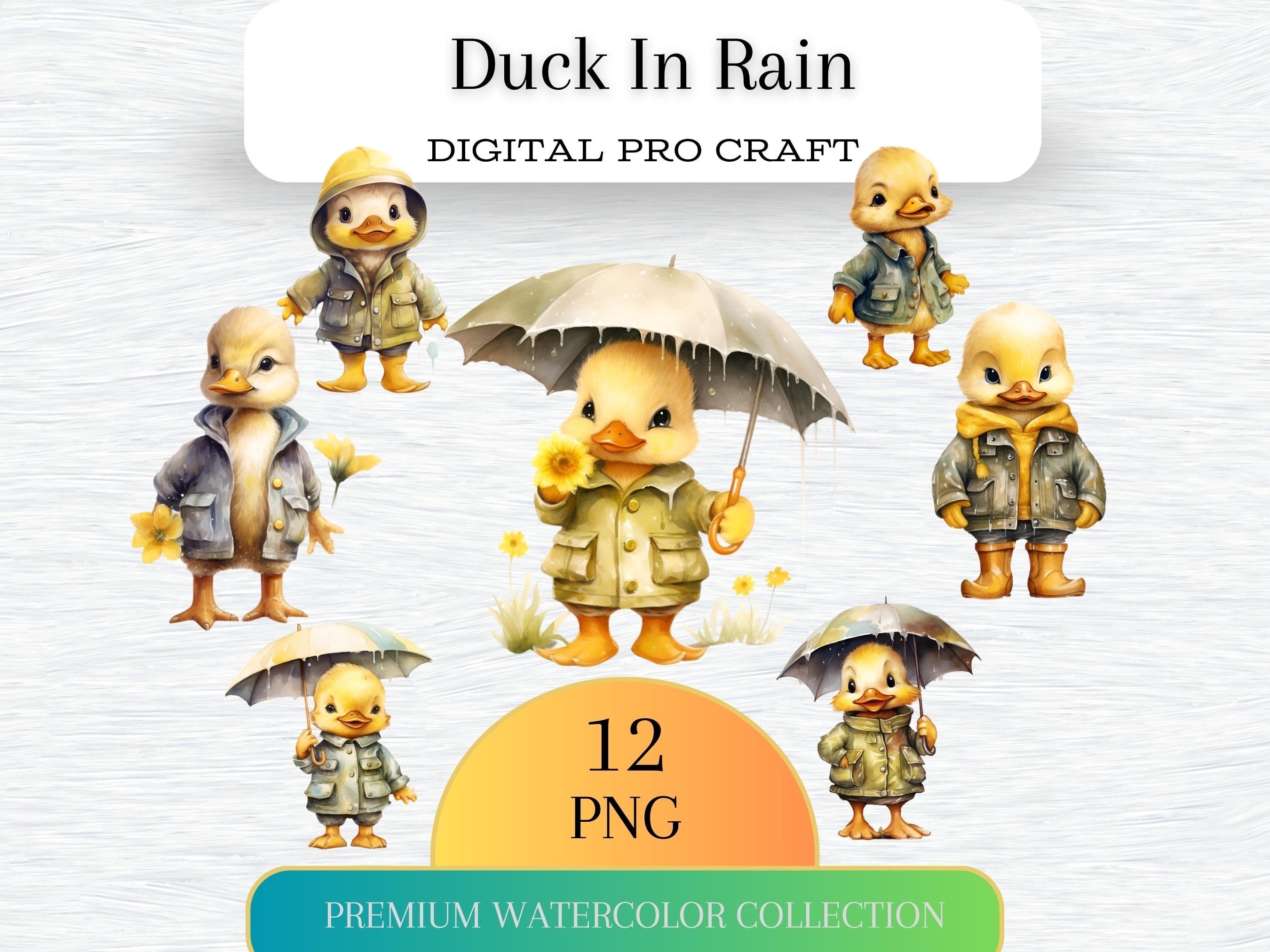The image showcases the front cover of a watercolor collection book titled "Duck in the Rain Digital Pro Craft." At the top, a prominent white banner with black text displays the title, with the first line in a huge font. Below this title, seven ducks are creatively arranged in a semi-circular pattern. The central figure is a duck adorned in a yellow rain jacket, holding a tan umbrella and a yellow sunflower. Surrounding this duck, other ducks exhibit unique attire: 

- To the left, a duck in a jean jacket is paired below with a larger duck in a jean jacket, yellow hoodie, and rain boots. Further below, another duck in a yellow puffer jacket holds an umbrella.
- To the right, starting from the top, a duck with a rain hat, raincoat, and yellow rain boots is seen. Below, a duckling in an open jean jacket holds a yellow flower in her right hand, and at the bottom, a duck in a jean jacket with four pockets carries an umbrella.

Underneath the central duck, an orange semi-circle features the text "12 PNG." At the very bottom, a blue banner reads "Premium Watercolor Collection." The vibrant, AI-created or painted ducks dressed in various rain gear add a playful touch to the cover's overall aesthetic.